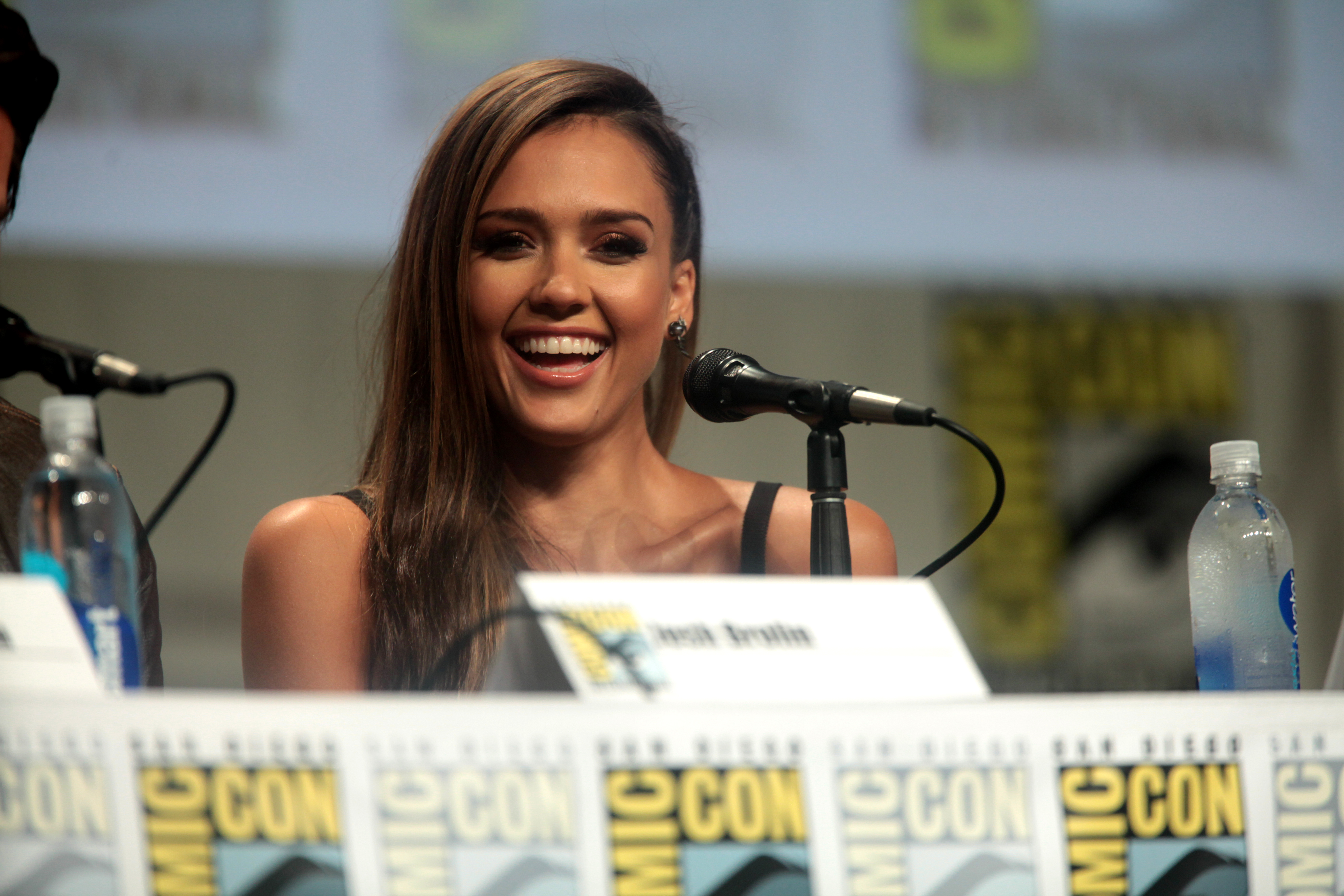In this horizontally aligned rectangular photograph, actress Jessica Alba is seated at a table at San Diego Comic-Con. She sits behind a black microphone on a stand, centered in the frame, with additional microphones visible near her and adjacent participants. Jessica is smiling broadly, revealing her teeth, and appears to be laughing. Her long brown hair cascades over her right shoulder, and she is wearing a black sleeveless top with visible straps. To her right, there is a water bottle with a blue label and a white cap—likely a chilled Smartwater bottle, as indicated by the condensation on its surface.

In the blurry background, there are large posters and a banner featuring the Comic-Con logo in alternating yellow and white squares. A similar banner drapes in front of the table, including a name card that, though it is indistinct, features her name and the Comic-Con icon. A shadow, possibly caused by a projector, is noticeable at the bottom of the image. Additionally, part of another person's shoulder and head can be seen to the left of Jessica, indicating she is amidst a panel of speakers.